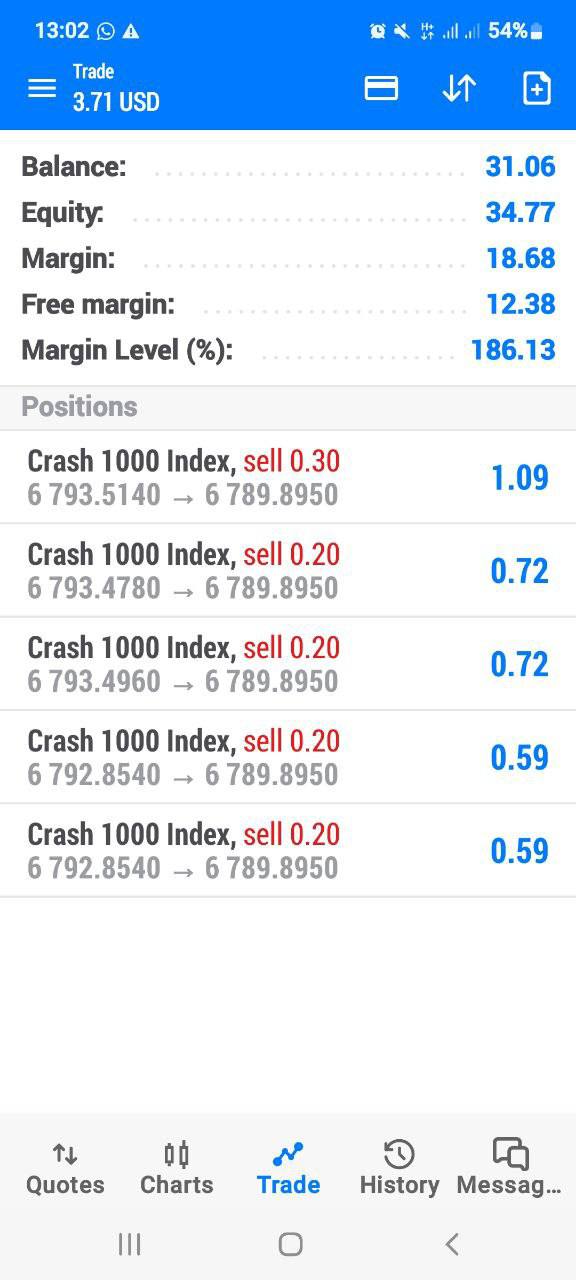The image displays a detailed view of a cellular phone screen, showcasing a financial trading application. At the top, the time is indicated as 13:02, with the battery level at 54% and the signal strength showing full bars. An alarm is set, confirming the device's concise setup.

The screen headline reads "Thomas's Trade," highlighted with various financial metrics:
- In red, a figure of $3.71 USD is prominently displayed.
- Below this, on a white background, are key account balances:
  - Balance: $3,106
  - Equity: $3,477
  - Margin: $1,868
  - Free Margin: $1,238
  - Margin Level Percentage: 186.13%

Also listed are specific trading positions:
1. "Crash 1000 Index Sell" with the values:
   - Position: 0.306
   - Current Value: 793.5140
   - Arrow to the right marking 6 spaces and another value: 789.8950
   - Market Value: $1.09
2. Another "Crash 1000 Index Sell":
   - Position: 0.206
   - Current Value: 793.4780
   - Right Arrow marking 6 spaces and another value: 789.8950
   - Market Value: $0.72

The screen appears to be very detailed, providing a comprehensive look at Thomas’s trading activities, balances, and ongoing market positions on the "Crash 1000 Index."